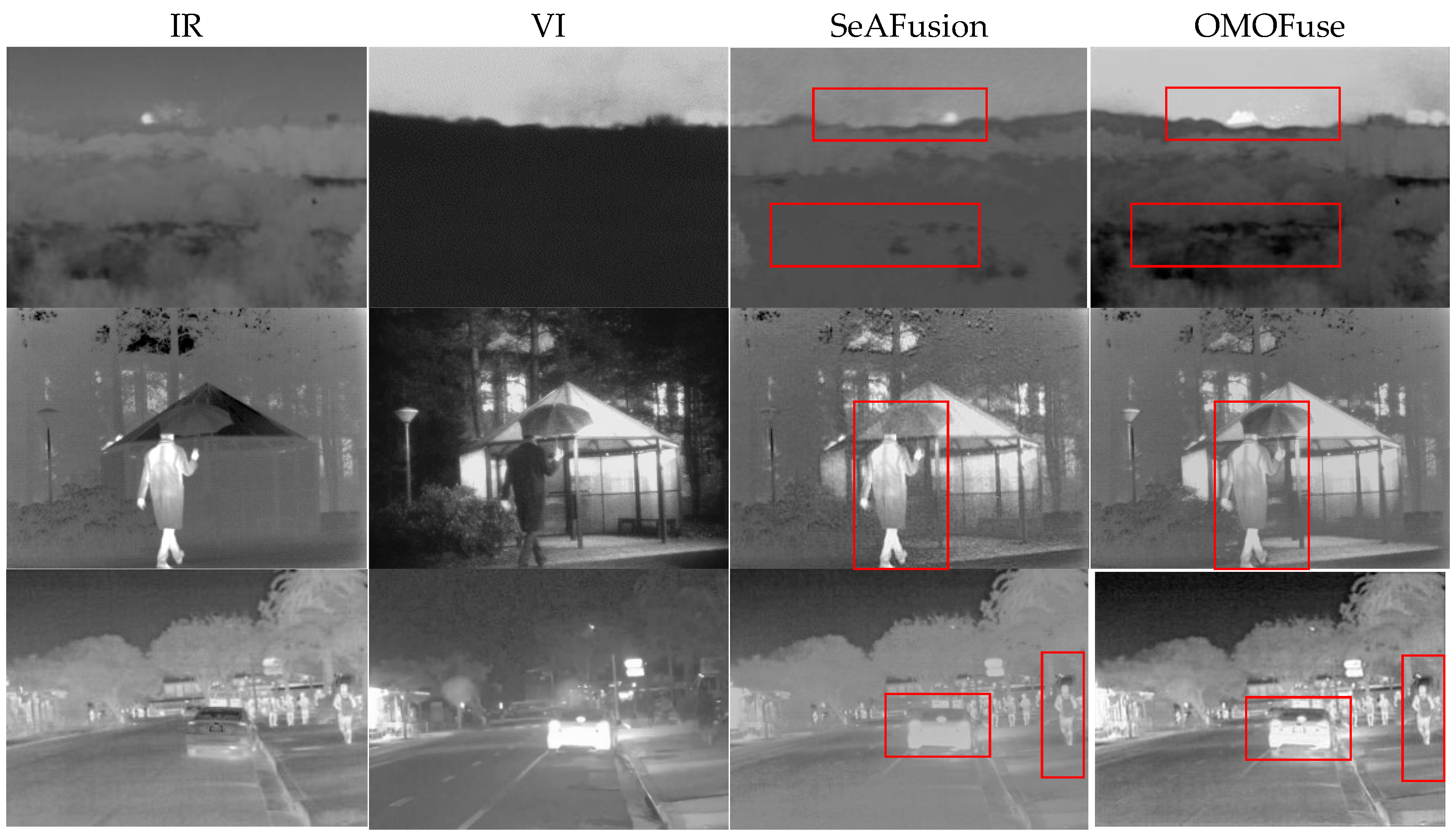The image displays a meticulously organized 3x4 grid of black and white photographs, each arranged in four vertical columns labeled respectively as "IR," "VI," "SEAFusion," and "OMOFuse." The photos exhibit various scenes, including a man walking with an umbrella on a road, a street view, a dense forest, and some snapshots containing vehicles and individuals. These photos are processed using different types of visual technologies, producing effects reminiscent of x-ray, night vision, and negative filters. Predominantly gray, black, and white in color, a few images are accentuated with red rectangle outlines, enhancing specific details. Overall, the photographs demonstrate how each technology uniquely interprets the same scenes, presenting distinct visual perspectives.